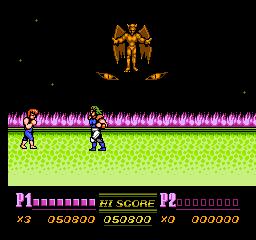This image is a screenshot from a handheld or arcade-style fighting video game. The top portion of the image has a black background with a menacing, brown-colored, winged gargoyle creature at its center. Below the gargoyle, two sinister, slanted eyes with yellow pupils peer out from the darkness, accompanied by tiny pinpricks of light resembling stars. The battleground below is a glowing green field, speckled with darker green spots and edged with a line of purple flames. On this field, two fighters stand ready for combat; the fighter on the left is in a boxing stance with raised fists, while the one on the right appears to be clad in silver armor and sporting green hair. At the bottom of the screen are the indicators "P1" and "P2," with corresponding purple square markers likely representing health or score. "P1" has several filled purple squares, whereas "P2" has outlined boxes, signifying their current status. A high score of 50,800 is prominently displayed at the center.